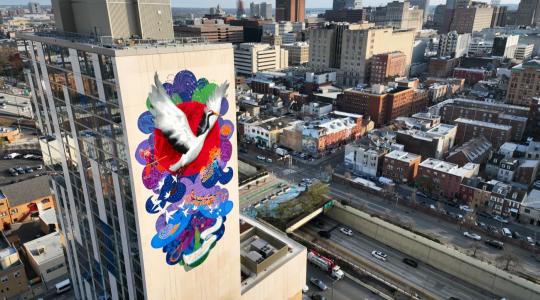This color photograph captures a bird's-eye view of an urban environment, taken from a significant height as if looking down from a tall building. Dominating the foreground in the bottom left is a tall, beige-colored building adorned with expansive glass windows on its left side. On the right facade of this building is a vibrant mural featuring what appears to be a stork or crane with a black head, white wings, and yellow beak, set against a bold red circle. Surrounding the bird are swirling blue and purple lines, and additional smaller birds, possibly doves, flying through the scene. Beneath and to the right of this building, the streets are bustling with cars, and shorter buildings are organized in square plots. In the distance, higher skyscrapers emerge, extending towards the top left and right of the image, with a hint of blue in the far center that might be either water or sky. The photograph, taken during the day, offers a detailed snapshot of the dynamic cityscape below.